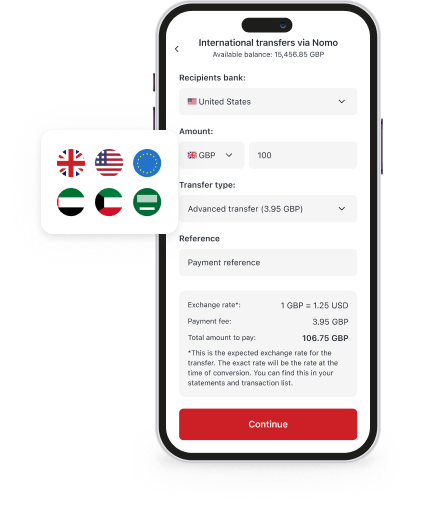A detailed and organized caption:

---

The image captures an ongoing attempt to transfer money via a mobile app. The focal point is a smartphone displaying the app's interface in portrait orientation.

At the very top of the screen, the app indicates the user is engaged in an "International Transfer via NOMO," with an available balance of £15,456.85 GBP. Below this, there's a section for the "Recipient's Bank," which specifies "United States" as the destination, accompanied by a dropdown menu for selection.

Further down, the "Amount" field allows for currency input, displaying an option for GBP with a dropdown, and next to it, another field shows "$100 USD." Below this, the "Transfer Type" is identified as "Advanced Transfer," incurring a fee of "3.95 GBP," again with a dropdown for additional options.

The next section includes a "Reference" field, currently filled with "Payment Reference" in a grey box. Below, the "Exchange Rate" is clearly stated, showing "1 GBP equals 1.25 USD." Additionally, the "Payment Fee" is reiterated as "3.95 GBP." The "Total Amount to Pay" is specified as "106.75 GBP."

A disclaimer indicates that the displayed exchange rate is expected for the transfer, but the exact rate will be determined at the time of conversion and can be found in the user's Statements and Transaction List.

A red "Continue" button with white text is located at the bottom of the screen, prompting the user to proceed with the transaction.

Outside the phone, towards the top left, there are icons of flags from Great Britain and several other countries, arranged in two rows of three within a square box.

---

This caption provides a comprehensive description of the image, detailing the interface and elements visible on the smartphone screen and some contextual elements positioned around it.